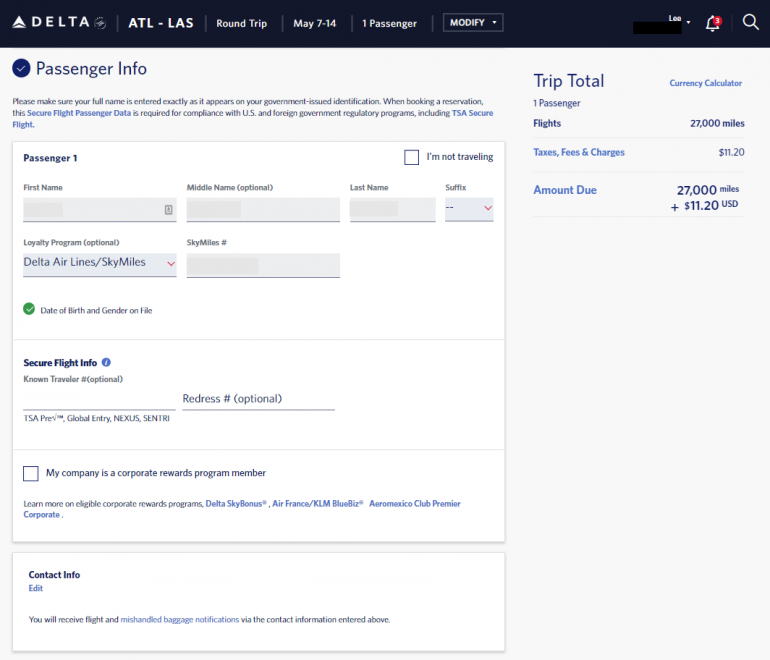This Delta Airlines webpage details a flight itinerary from Atlanta (ATL) to Los Angeles (LAS). At the top left, the Delta logo is prominently displayed, featuring a white triangle with a small bottom segment separated, alongside "DELTA" in all caps. Next to the logo, the flight details "ATL-LAS" are listed. Below, a dark blue navigation bar with grey separators includes options: "Round Trip," "May 7th to 14th," "One Passenger," and a drop-down menu for currency.

On the right side of this bar, the page shows a blurred-out passenger name next to "Lee," accompanied by a bell icon indicating three notifications with a red circle and white text, and a white magnifying glass icon for search functionality.

Below this bar, "Trip Total" is displayed in dark blue, adjacent to a lighter blue text mentioning "Currency Calendar." The booking details highlight "One Passenger" and list available flights. To the right, it mentions a total of "27,000 miles" and provides a link ("Terms, Fees, and Charges") indicating an additional cost of $11.20. The segment confusingly mentions "Mountain Dew" alongside a repeated cost summary of "$27,000 plus $11.20 USD," likely a miscommunication in the voice capture.

On the left side, there's a "Passenger Info" section featuring input fields for the first, middle, and last name, suffix, and Delta loyalty program membership (SkyMiles). However, the SkyMiles number is not displayed. At the bottom, "Contact Info" is highlighted in dark blue with an "edit" link for modifications.